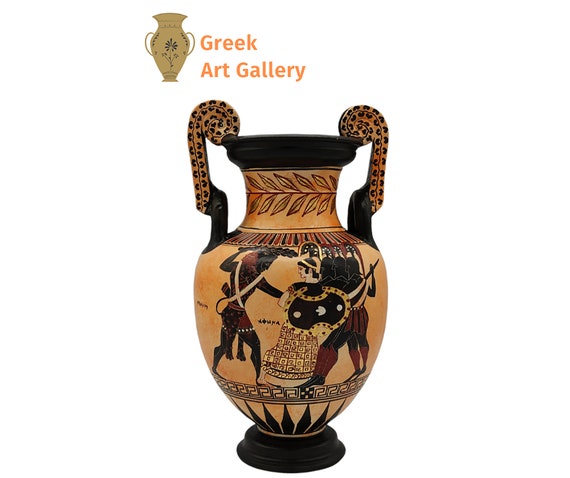The image features a large, vertically oriented Greek vase with two ornamental scrolled handles on either side, set against a white background. Crafted in a classic black and orange color scheme, the vase showcases intricate decorations from ancient Greece. The main motif includes mythical figures and Spartan warriors, with a central seated woman adorned with a shield and helmet, while a man holding a branch stands on the left. Additional warriors are depicted in the background. The neck of the vase is encircled by an elegant leaf pattern, and the base features dark black geometric designs rising upwards. The top and bottom sections of the vase are solid black. A watermark at the top includes a small, generic vase illustration and the words "Greek Art Gallery" in green. The vase rests on a pedestal, enhancing its timeless and artistic appeal.